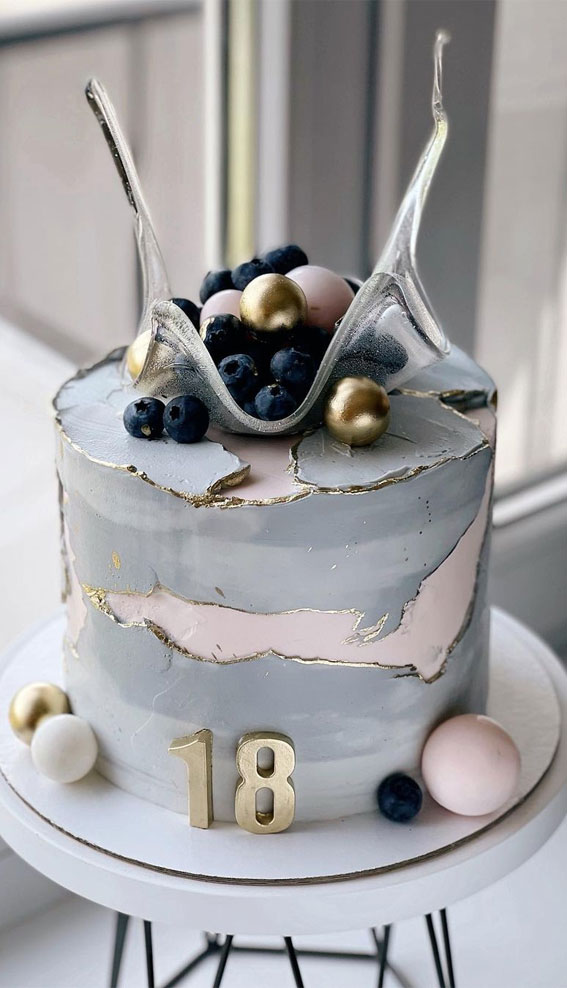This full-color indoor photograph, staged with natural light, showcases an elaborate birthday cake standing on a round white pedestal with visible black metal legs. The vertically rectangular image features a visually striking cake, approximately 10 inches tall, predominantly in steel blue with sections that appear artistically shattered to reveal a pale pink inner layer framed by golden edges. Adorning the top of this unique confection are clusters of blueberries and an elegant, transparent pulled sugar sculpture that adds a sophisticated touch. Throughout the cake, decorative globular objects can be found, including three gold spheres, two larger pink ones, and additional blue and black ones. Towards the center bottom of the image, about 25% up from the base, a bold gold number "18" is prominently displayed, signifying the birthday celebration.